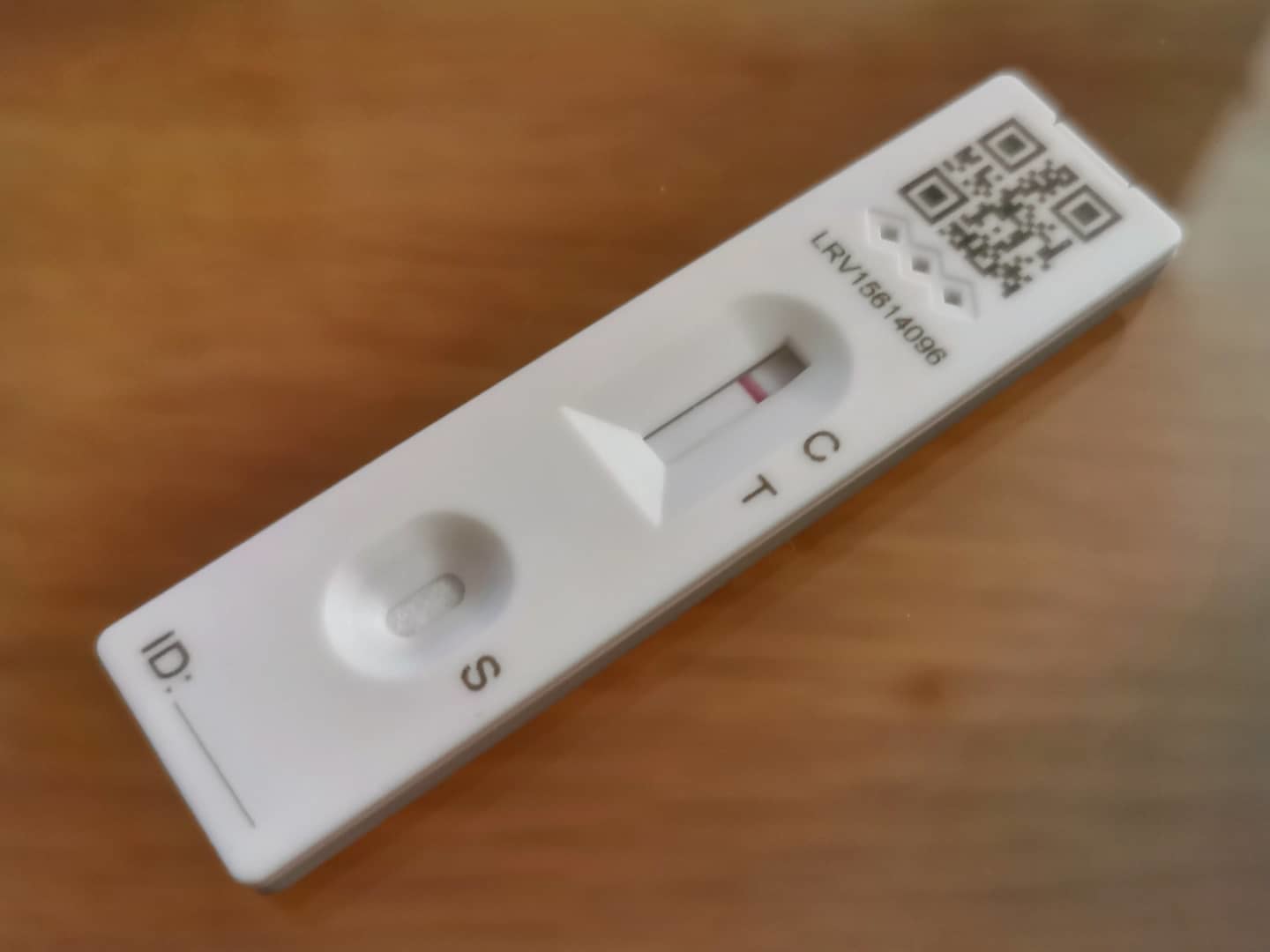A close-up image of a COVID-19 test strip is displayed on a brown wooden table. At the top of the test strip, a barcode is visible, followed by the alphanumeric code "LRV15614096." Below this code, the control (C) and test (T) areas are marked, with a red line appearing next to the control (C), indicating that the test is working correctly. The test line (T), which would indicate the presence of the virus, is blank, suggesting a negative result. At the bottom of the test strip is an oval section labeled with an "S," where the sample would be applied. Additionally, there is an ID section with a blank space next to it for identification purposes. The entire test strip rests on a brown wooden table, providing contrast against the neutral backdrop.